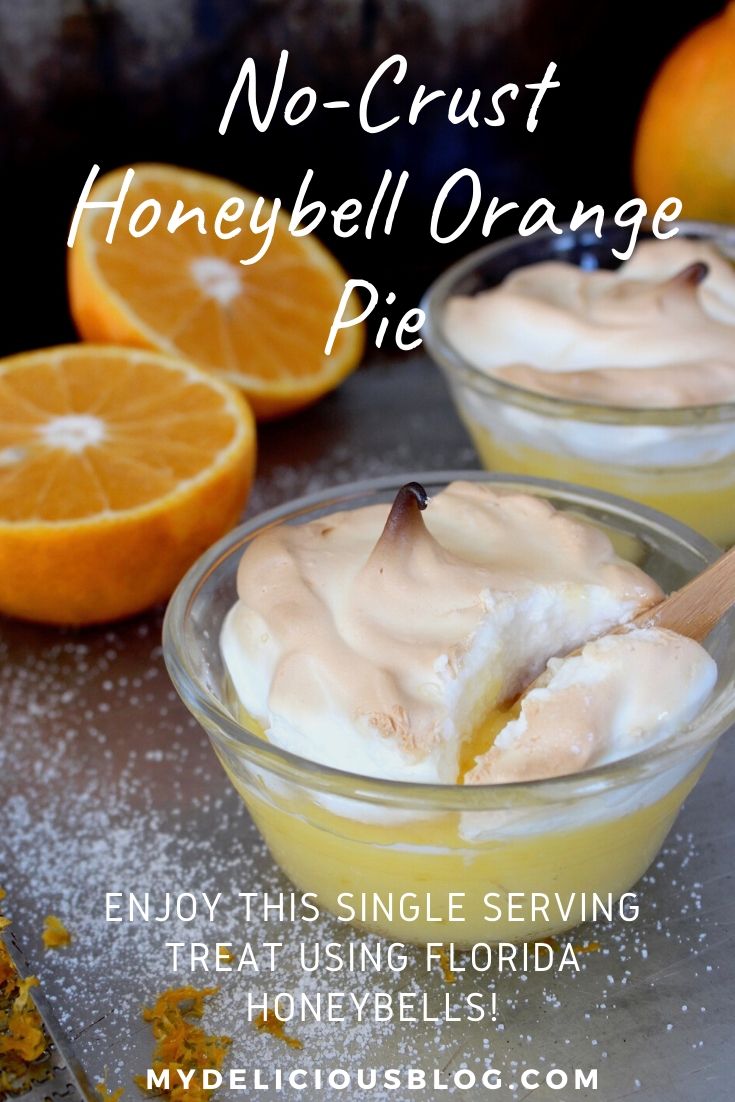The image features a visually appealing "No-Crust Honey Bell Orange Pie," as stated in a white, handwritten-style font at the top against a black background. The scene is set on a gray, metallic surface sprinkled with sugar and orange zest. In the foreground, there are two glass bowls, each filled with a vibrant yellow filling and topped with a perfectly browned meringue. A wooden spoon is seen dipping into the front bowl, adding a touch of rustic charm. In the background, three oranges are positioned: on the left, an orange is halved, revealing the juicy interior, while on the right, a whole orange is slightly out of focus. The text at the bottom invites viewers to "Enjoy this single serving treat using Florida Honey Bells," with the website MyDeliciousBlog.com prominently displayed. White specks are scattered throughout, enhancing the festive and inviting atmosphere of the image.